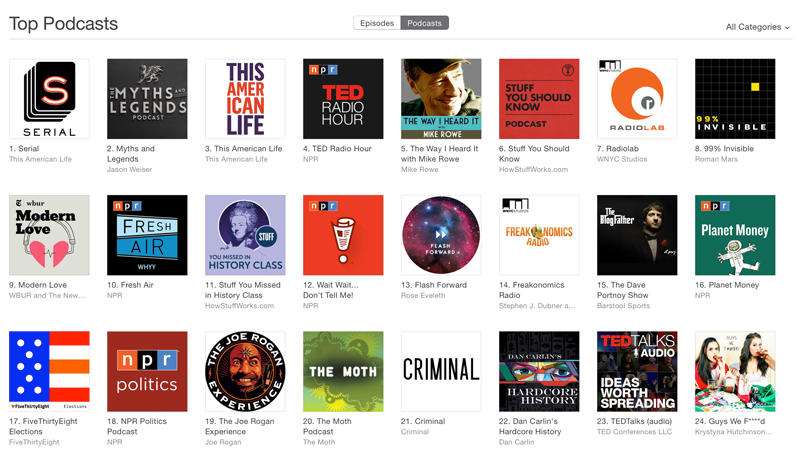A horizontal image showcases a white background featuring a web page listing the top podcasts. The top left corner prominently displays the label "Top Podcasts." At the center of the page, two sections are highlighted: "Episodes" and "Podcasts." On the top right corner, there is an option labeled "All Categories."

The list begins with:

1. Serial
2. Myths and Legends
3. This American Life
4. TED Radio Hour
5. The Way I Heard It with Mike Rowe
6. Stuff You Should Know
7. Radiolab
8. Invisibilia

The list of podcasts continues up to 24 entries in total.

Each podcast is represented by an 8x3 grid of square icons, each resembling an album cover or logo that includes brief descriptive text. Noteworthy podcasts on the grid include:

- **Second Row:** Modern Love, Fresh Air, Stuff You Missed in History Class, Wait Wait... Don't Tell Me!, Flash Forward, Freakonomics Radio, The Dave Portnoy Show, Planet Money
- **Subsequent podcasts:** FiveThirtyEight Elections, NPR Politics Podcast, The Joe Rogan Experience, The Math Podcast, Criminal, Dan Carlin's Hardcore History, TED Talks, Guys We F****d.

The page visually arranges these icons from left to right and top to bottom, offering users a comprehensive, organized view of popular podcasts.